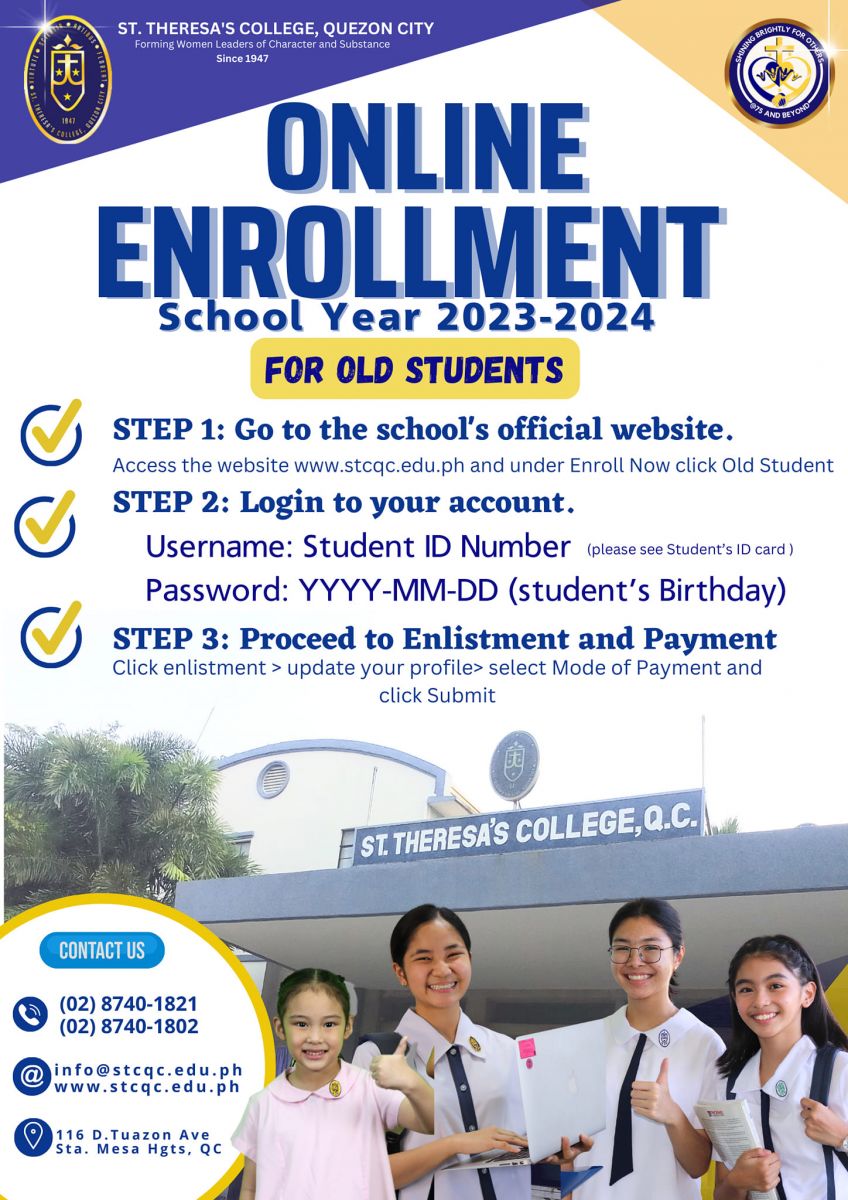A promotional flyer from St. Teresa's College in Quezon City showcases the institution's commitment to "Forming Women Leaders of Character and Substance Since 1947." The flyer features the school's coat of arms, which includes a cross, highlighting its Catholic roots. The flyer announces "Online Enrollment for the School Year 2023-2024" with a special note in a bright yellow banner stating "For Old Students," indicating a streamlined enrollment process for returning students. 

The detailed steps for enrollment are outlined as follows:
1. Go to the school's official website.
2. Log in to your account.
3. Proceed to enlistment and payment.

The flyer also features a joyful image of four young girls in school uniforms, smiling, likely representing the inclusive and vibrant student community. Essential contact details, including a phone number, email, and the college's location, are provided to assist with any inquiries. The imagery and content suggest a warm, welcoming environment that values tradition and character-building education in the Philippines.